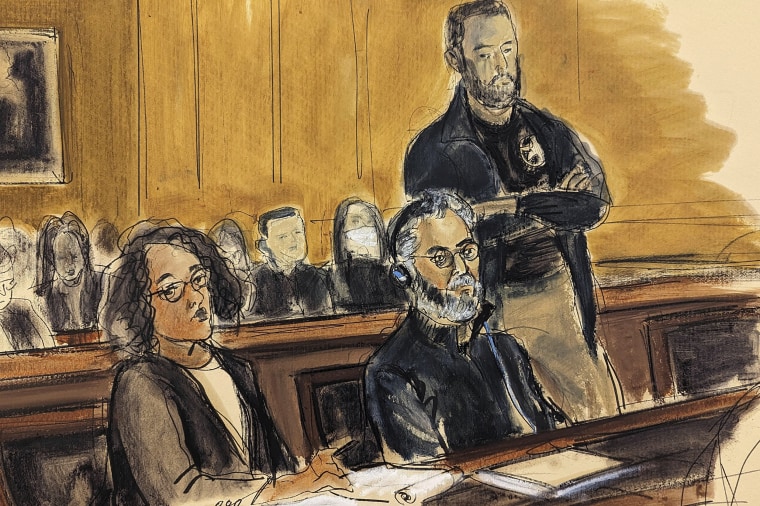In this detailed color courtroom sketch, the scene captures a solemn courtroom proceeding. At a wooden-paneled bench, a dark-skinned woman with shoulder-length black hair, wearing glasses and dressed in a black suit with a white shirt, sits attentively with her hand poised over a legal pad. To her right, an older man, likely in his late 50s or early 60s, sits wearing a black long-sleeved button-down shirt. The man has whitish-gray hair with traces of salt and pepper, wears round glasses, and has full facial hair. Notably, he has headphones on and a pad in front of him.

Standing directly behind this man is a court bailiff, characterized by his close-cropped hair, full facial hair, and a sheriff's badge prominently pinned to his uniform. He stands cross-armed, gazing down at the man seated at the desk.

In the background, a jury is seated, with one of the jurors notably wearing a COVID mask. Observers form a backdrop behind the main figures. The courtroom’s decor includes a painting on the wall, adding to the formal atmosphere of the judicial setting.